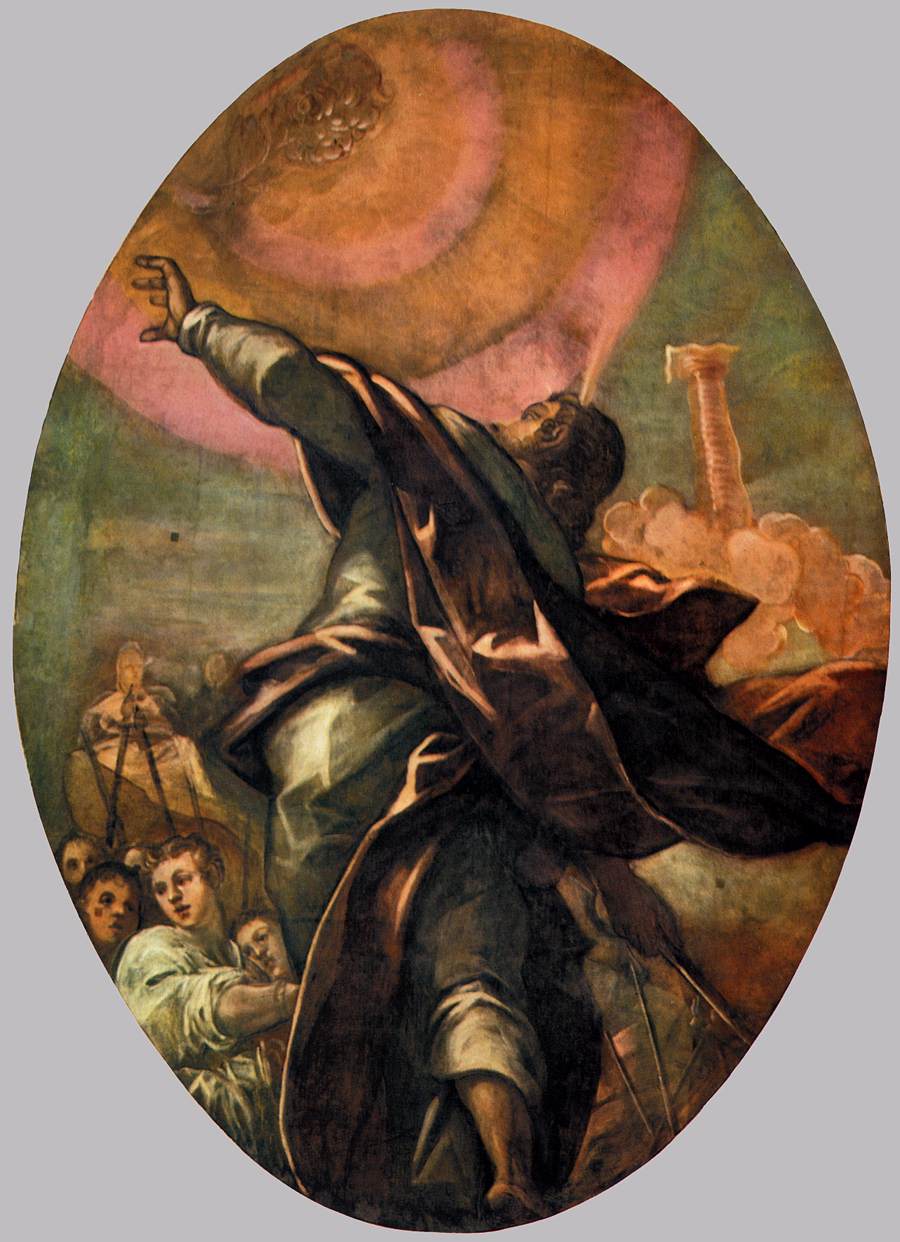This painting, elegantly set within a vertically oriented oval frame against a contrasting gray rectangular backdrop, vividly depicts a scene that exudes a mystical and ethereal quality. Dominated by a palette of olive, orange, and pink hues, the artwork features a central figure—a man draped in a long white gown interwoven with an orange sash—reaching upward towards the heavens with his left arm. His posture and barefoot state, along with his long flowing hair, hint at a sense of ascension or divine calling. Above, vibrant rings of orange and pink create a celestial ambiance, possibly indicating a heavenly presence or divine light.

Beneath this uplifting scene, the lower portion of the painting portrays a small gathering of people in the bottom left. Among them, a couple of individuals gaze at the ascending figure while others seem entranced by different focal points. The detailed expressions and postures suggest varied reactions to the central man’s heavenly reach. In the sky, to the right side beside the ascending man, an indistinct figure or possibly an angel can be seen through wisps of an orange cloud, adding to the painting's divine narrative. The overall composition skillfully balances the mystical ascent with the earthly spectatorship, merging human devotion and celestial elevation.